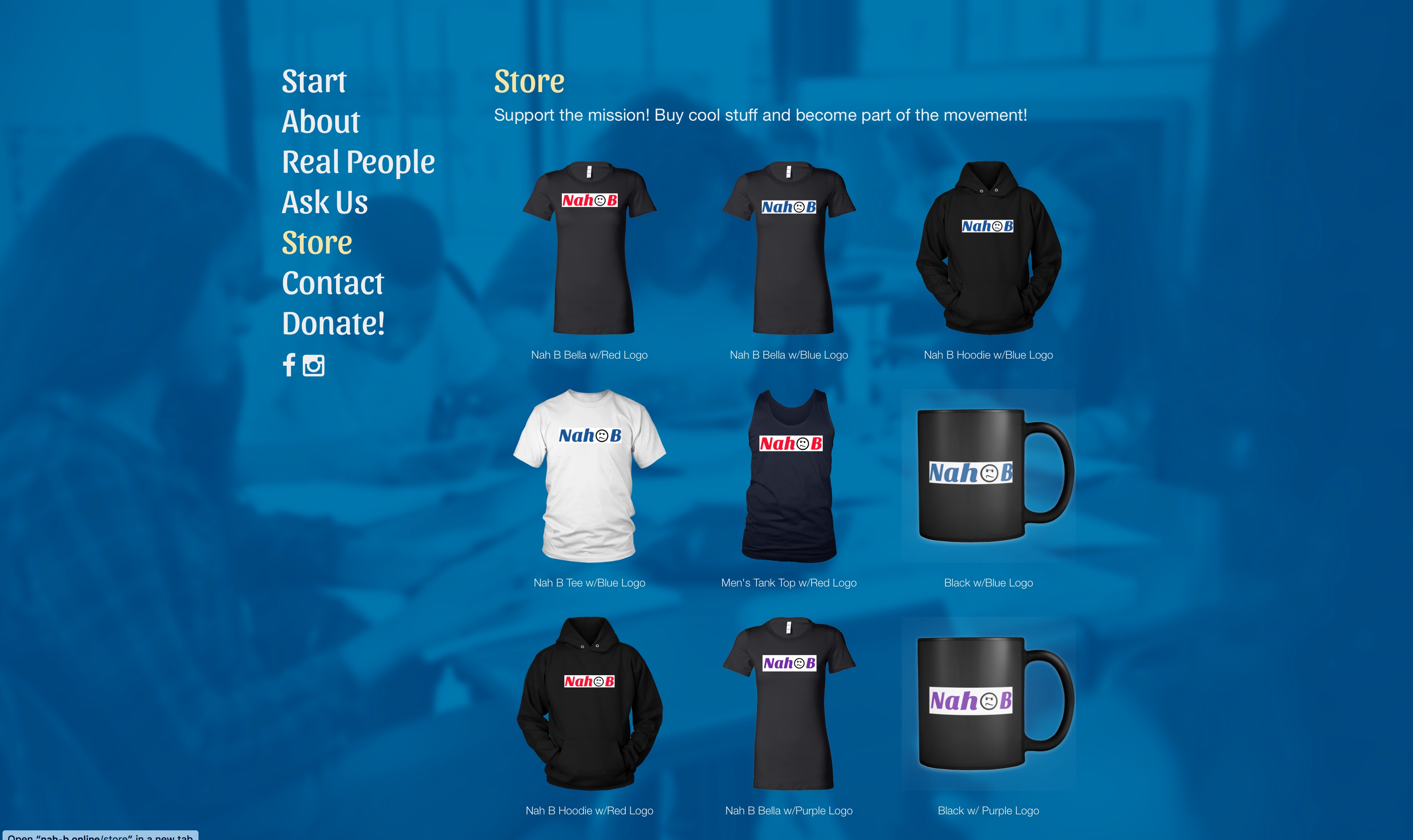Screenshot of an online storefront showcasing various merchandise. The page features navigation options such as Start, About, Real People, Ask Us, Store, Contact, and Donate, alongside Facebook and Instagram icons for social media connectivity. The currently selected option is "Store," which appears in the left sidebar. Centered in the middle is a background image depicting individuals collaborating on ideas.

Underneath the "Store" heading, motivational text reads: "Support the mission, buy cool stuff, and become part of the movement." Displayed products include:

- A black hoodie
- Two black T-shirts bearing the design "Nah-B." The design features the letters "N-A-H," a smiley face, and the letter "B."
- Various items such as T-shirts, hoodies, tank tops, and coffee mugs exhibit diverse color schemes, with logos in red, blue, and purple.

Product descriptions include:

- "Nah-B Bella T-shirt with red logo"
- A hoodie with a blue logo
- A coffee mug with blue lettering
- A tank top with a red logo
- An all-black coffee mug with purple lettering
- A Nah-B hoodie with red lettering

These items are prominently displayed, inviting viewers to support the cause through their purchases.